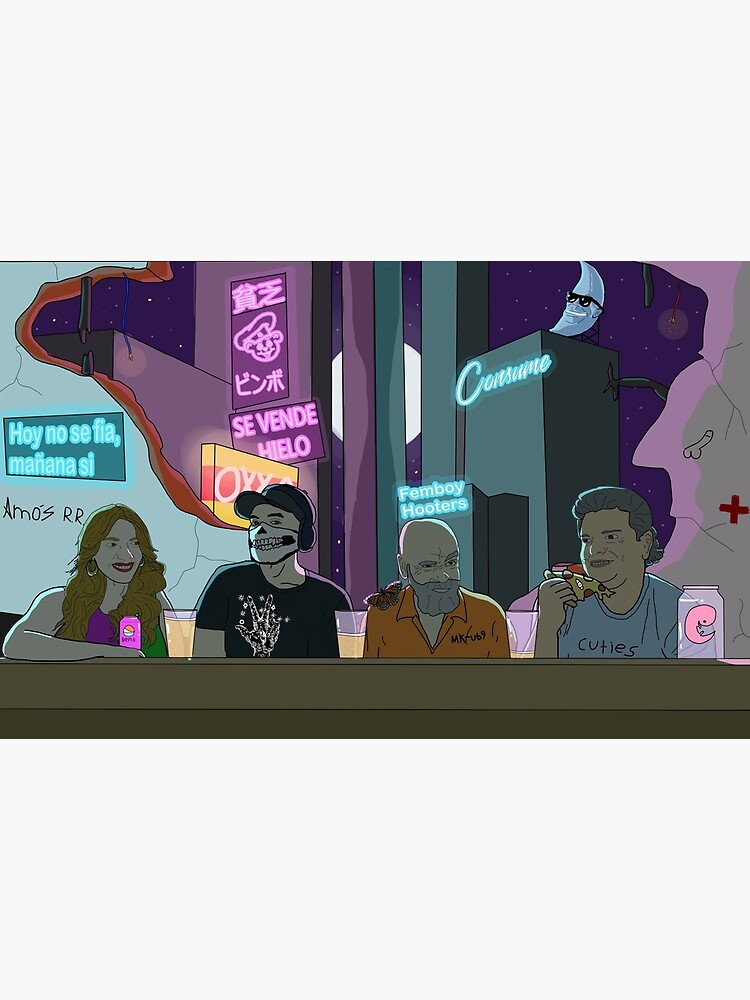A detailed cartoon drawing depicts a diverse group of four individuals seated at a bar or diner, set against a striking backdrop featuring a giant hole in the wall. Through this opening, a bluish-purple night sky with a moon bearing a face and glasses is visible amidst a cityscape adorned with neon logos such as "Vindy Hello" and "Femboy Hooters." Inside the scene, illuminated signage reads, "Hoy no se via, Mediana Si," adding to the vibrant atmosphere. 

Starting from the left, a blonde-haired woman with white skin dons a pink shirt and holds a pink drink. Beside her, a man in a black shirt with a peace sign graphic sports a cap and a face mask depicting frightening teeth. Next is an older man with a beard and mustache clad in an orange prison jumpsuit, distinguished by a butterfly on his shoulder. On the right, another figure with gray hair and a light blue shirt featuring the word "Cuties" enjoys a slice of pizza, with a drink or small figure inside a jar nearby. The bar scene, laden with neon lights and graffiti, hints at an adult-oriented, bustling nightlife in an urban setting.